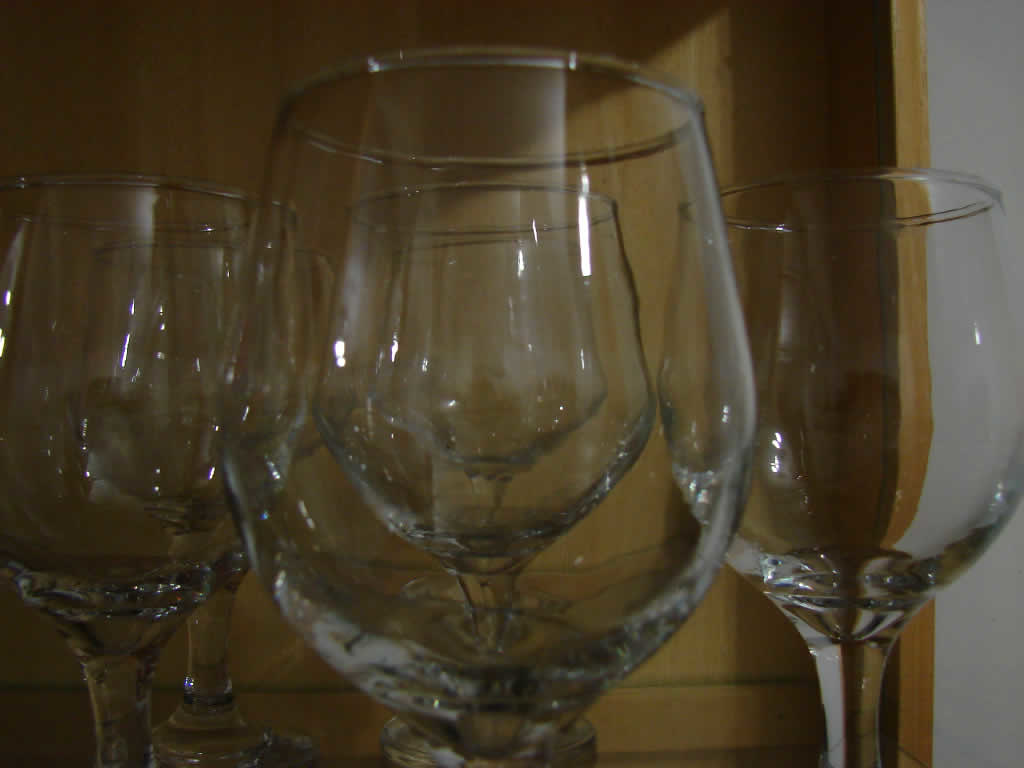The photograph captures a neatly organized wooden kitchen cabinet, crafted from oak, with its door open and light illuminating the scene from the right side. Inside the cabinet, there are at least six to seven long-stemmed, clear crystal wine glasses, meticulously arranged. The glasses are clean and reflect the surrounding light, showcasing their smooth and elegant design. Each stem has an intricate shape or design where it meets the cup. Adjacent to the cabinet, the right wall is white, enhancing the clarity and brightness of the image. These high-quality glasses are perched upright on the shelves, emphasizing their pristine condition and the orderly nature of the setting.